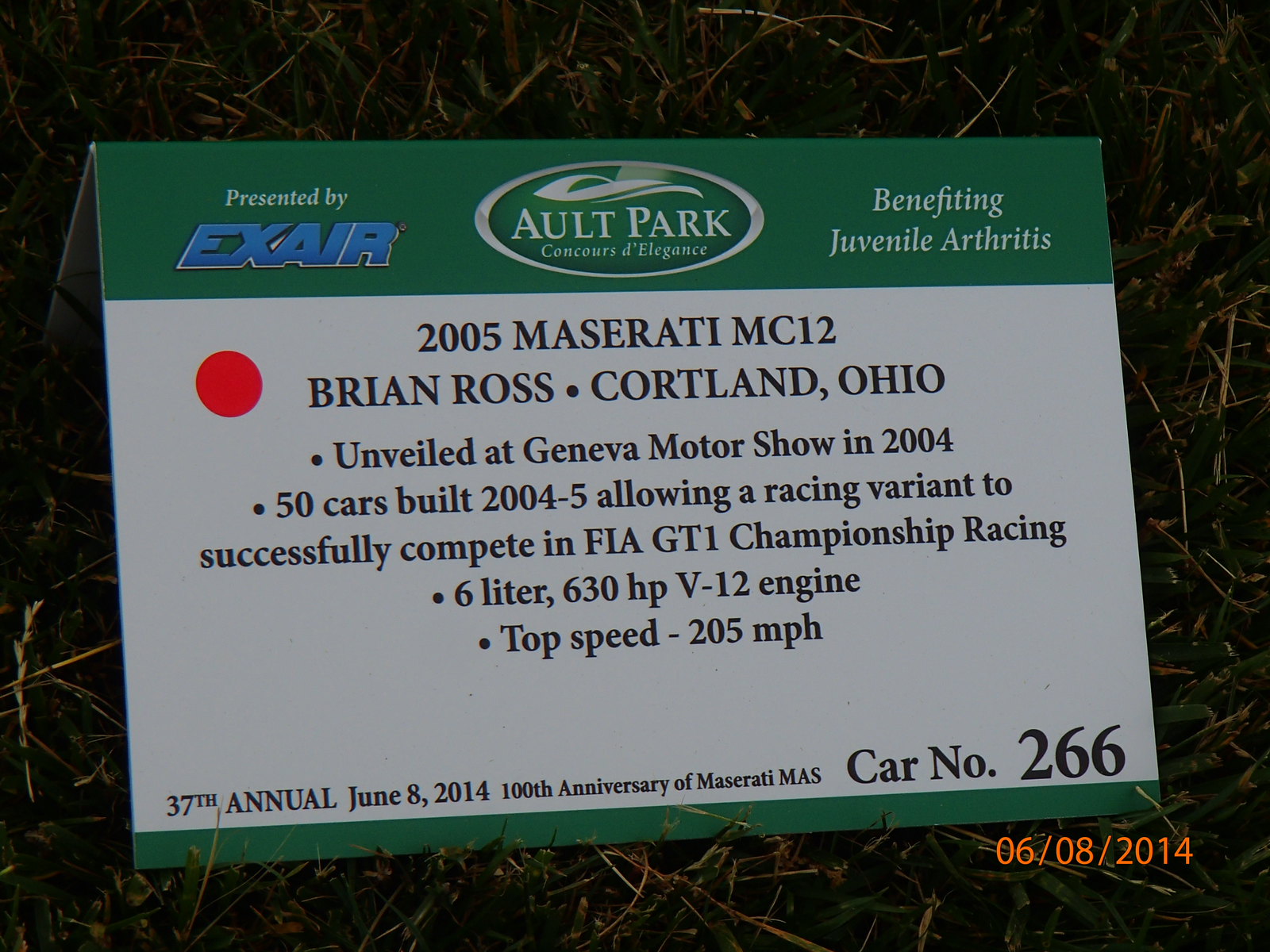The image features a detailed sign positioned on dark, patchy grass. The sign is primarily white with dark green sections at the top and the bottom. The top section prominently displays the words "AULT Park Concours d'Elegance," encircled in an oval. On the left, it reads "Presented by AXA," and on the right, "Benefiting Juvenile Arthritis." The central white area of the sign provides detailed information about a significant automobile: a 2005 Maserati MC12. It notes that this model was first unveiled at the Geneva Motor Show in 2004, with only 50 cars built between 2004 and 2005, designed to compete successfully in FIA GT1 Championship Racing. It highlights the car's specifications, including a 6-liter, 630 HP V12 engine and a top speed of 205 miles per hour. Additional text underscores the occasion — the 37th annual event on June 8th, 2014, celebrating the 100th anniversary of Maserati, noting this particular car as number 66. The sign sits against a background with some brown, dead grass and shrubs visible around its borders.